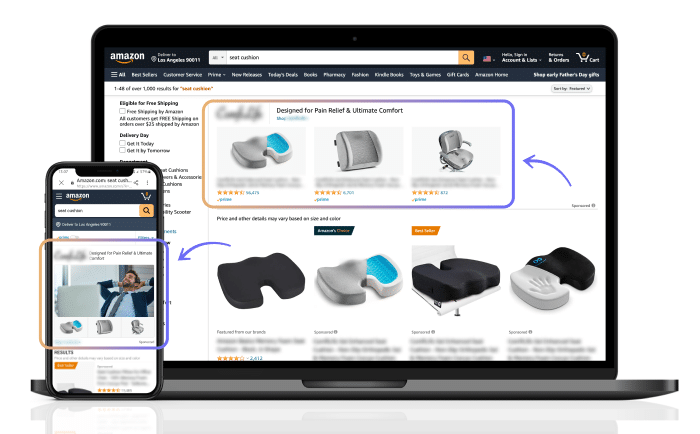The image displays an Amazon search page featuring a comparative infographic illustrating how the product listing appears on both a computer and a mobile device. The infographic prominently highlights a seating cushion and a neck pillow designed for pain relief and ultimate comfort. On the left side, a man is shown on a mobile device, relaxing with his hands behind his head. The right side showcases detailed product images of the cushion and pillow, emphasizing their ergonomic design. The Amazon logo is prominently displayed in the top left corner. The product, available in black and white, aims to enhance seating comfort, whether used as a cushion for chairs or as a supportive back pillow.